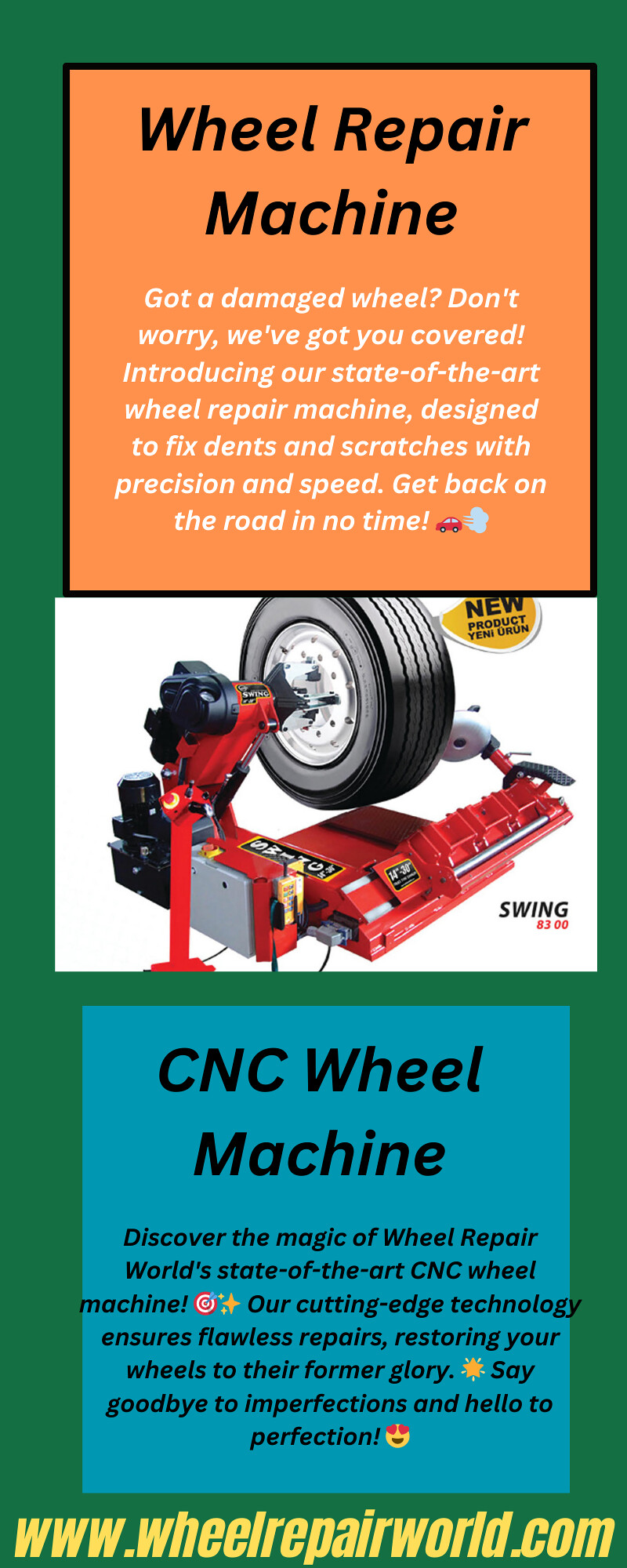This detailed advertisement for Wheel Repair World features a vertically oriented design divided into three main sections, all set against a dark green background. At the top, a rectangular box with a peachy-orange background presents the header "Wheel Repair Machine" in bold black letters. Beneath this header, white text elaborates on the service: "Got a damaged wheel? Don't worry. We've got you covered. Introducing our state-of-the-art wheel repair machine designed to fix dents and scratches with precision and speed. Get back on the road in no time." This section also includes a small graphic of a car and mechanic.

The middle section features a white background and displays an image of a red wheel repair machine working on a floating black tire, illustrating the product in use. This section is meant to visually demonstrate the functionality of the machine.

The final section at the bottom is a teal-colored rectangle with "CNC Wheel Machine" boldly written in black text at the top. Beneath this, another paragraph details the CNC wheel machine service: "Discover the magic of Wheel Repair World's state-of-the-art CNC wheel machine. Our cutting-edge technology ensures flawless repairs, restoring your wheels to their former glory. Say goodbye to imperfections and hello to perfection." This section is accented with an emoji to emphasize satisfaction.

At the very bottom of the advertisement, the website www.WheelRepairWorld.com is displayed in yellow italics against the green background, guiding viewers on how to find more information.